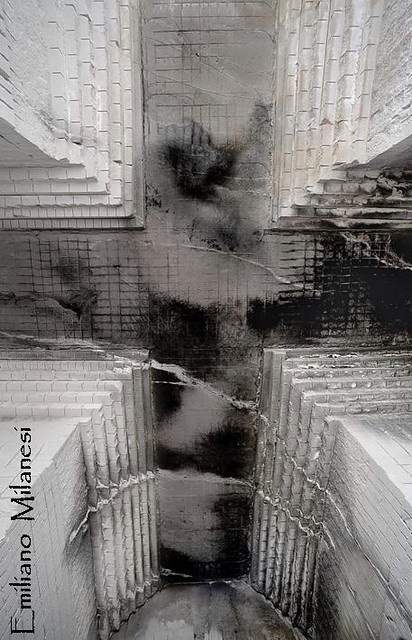This black-and-white abstract artwork, created by Emiliano Milanesi, presents a complex, mesmerizing view that can be interpreted in multiple ways. The image possibly depicts an aerial perspective of intersecting buildings or an intricate intersection of columns viewed from either above or below. Throughout the composition, there are repeated elements of thick, white bricks forming chunky, layered structures resembling steps or tiled surfaces. 

The top left and right corners, as well as the bottom edges, feature these stepped, tile-like formations, framing a central area that takes on a cross shape. The middle section is characterized by flat gray tiles interspersed with irregular black splotches and intersecting gray and white lines that extend across the painting, creating an intricate network of patterns. The black patches are more concentrated on the right and lower sections, adding a sense of depth and complexity, while cracks traverse the image, adding a dynamic, almost fractured appearance.

Near the bottom left corner, the artist's name, "Emiliano Milanesi," is subtly integrated into the design, providing a signature to this visually stimulating and thought-provoking piece. The image challenges the viewer's perception, offering a different interpretation with each glance, making it a captivating example of modern abstract art.